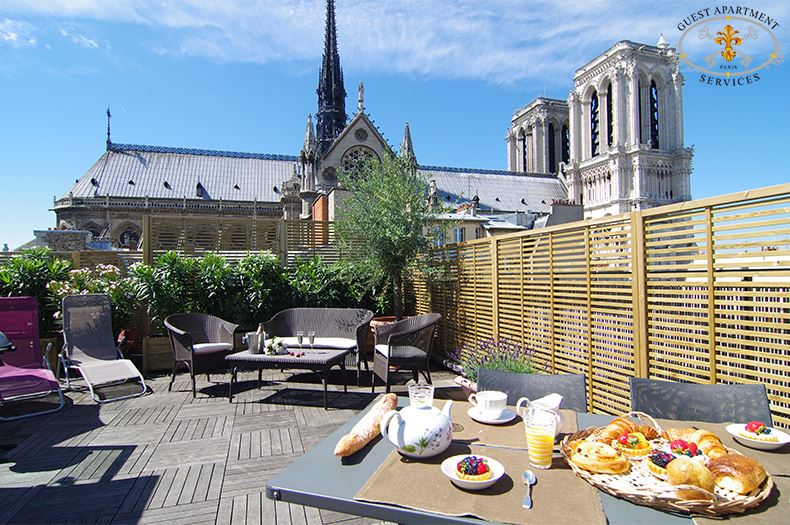The image depicts an outdoor dining area on the rooftop patio of a hotel facility, likely in Paris, France. The scene unfolds under a beautiful blue sky, with the intricate, castle-like features of Notre Dame Cathedral providing an iconic backdrop. The patio, surrounded by a brown, slatted wooden fence and decorated with wooden planter boxes filled with lush green bushes and a large potted plant with a small tree, exudes a serene ambiance. The flooring is composed of dark brown wood-like tiles.

In the foreground, the bottom right corner features a table set for guests, adorned with a tray of pastries, including croissants and fruit tarts, as well as a baguette, a white teapot, plates, and an assortment of fresh fruit. The table is further complemented by beige placemats and gray surface detailing. Additionally, an ice bucket with a bottle and two wine glasses is visible on another table towards the back. Comfortable patio furniture, including lounge and bench-type chairs, is arranged invitingly around the deck.

In the upper right corner of the image, there is an elliptical logo with "Guest Apartment Services" written around a central gold fleur-de-lis, further hinting at the luxury and attention to detail this establishment offers its guests.